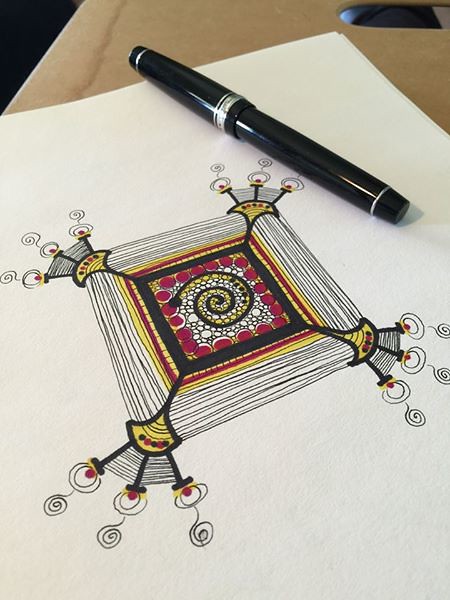The image portrays a white sheet of paper set against a tan or light brown desk. Sprawled across most of the paper is an intricate, square-shaped drawing created predominantly in black ink, with accents of red, yellow, and purple. The design features a variety of geometric shapes including squares, circles, and spirals, and resembles a mathematical or mandala-like pattern. Each of the four corners of the square is adorned with a spiderweb-type design, featuring fan-shaped clusters of thin lines that encircle small spirals. Dotted around these elements are small circles and swirls, contributing to the overall detailed complexity of the artwork. Lying almost diagonally in the upper right-hand corner of the paper is a black and silver pen, enhancing the artistic theme of the scene. The image is devoid of any readable text, allowing the elaborate pen-drawn artwork and the well-coordinated pops of color to capture the viewer's attention.